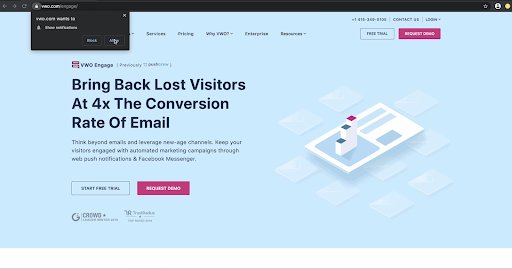The image is a screen capture from a website, featuring a web browser window with a black address bar at the top. In the address bar, a web address is typed out next to a padlock icon, indicating a secure connection. On the left side of the address bar, there are grayed-out navigation buttons including a back arrow, forward arrow, and a home button. On the right side, there's a star icon and a circular user icon with a black silhouette inside and a yellow dot.

Below the address bar, a black pop-up box with white text appears, featuring two buttons labeled "Block" and "Allow." The mouse cursor is positioned over the "Allow" button.

The website content itself has a light blue background with black text and various interactive elements. Prominently displayed towards the center is a message stating, "Bring back lost visitors at four times the conversion rate of email." Beneath this, a call to action encourages visitors to "Start free trial," and another box marked "Request demo" is highlighted in pink and white.

Additionally, a section at the bottom highlights various companies endorsing the product. To the right, there is an illustration of a white ID card featuring graphical elements, including graphs in blue and pink, and several white squares in the background, adding to the visual complexity of the page's design.